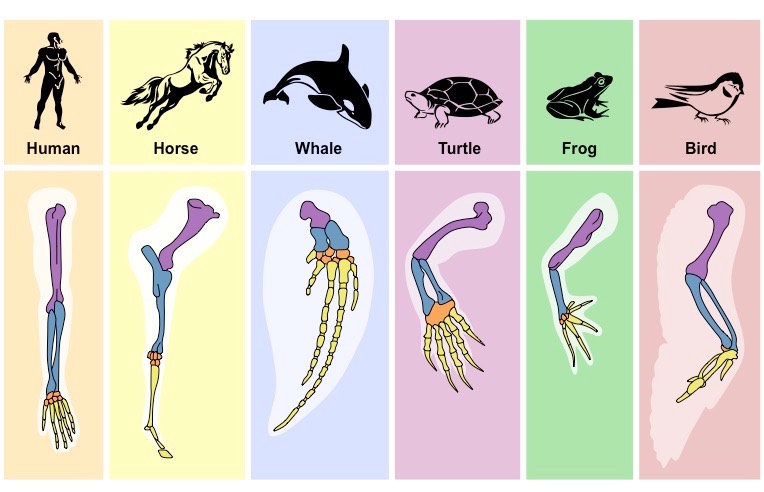The image is a detailed and colorful chart depicting the limbs of six different animals: a human, horse, whale, turtle, frog, and bird. Each animal is represented in its own vertical section, with the top portion featuring a simple black silhouette of the animal set against a uniquely colored background for easy identification and differentiation. Below each silhouette is a corresponding detailed diagram of the animal's limb bones, rendered in vivid colors—purple, blue, orange, and yellow—highlighting various parts of the bone structure. Human limbs are displayed in yellow background panels, horses in blue, whales in white, turtles in purple, frogs in green, and birds in pink. Detailed annotations of the bones, such as the femur and metatarsals, are meticulously illustrated, emphasizing the similarities and differences in limb anatomy across these species. Overall, the chart provides a comprehensive and visually engaging comparison of the skeletal structures of each animal's limb.